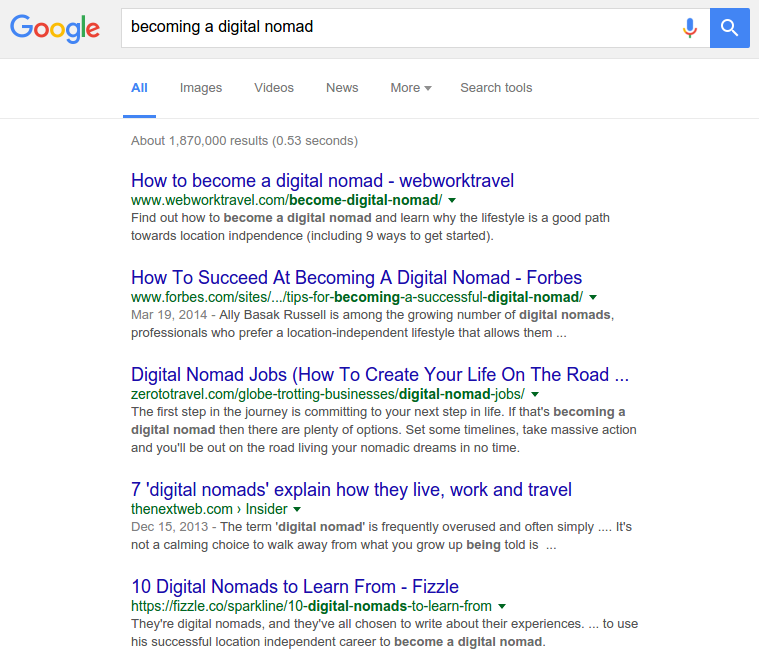The image displays a Google search page with a white background. In the top left corner, the search bar shows the query "becoming a digital nomad." Below the search bar are various tabs such as All, Images, Videos, News, and Search Tools, with the "All" tab highlighted in blue. Underneath, there is a grey text stating, "About 1 million internet and 70,000 results in 0.53 seconds."

Five search results are prominently shown:

1. **Title**: How to Become a Digital Nomad - Web Travel  
   **URL**: [webtravel.com](http://webtravel.com)  
   **Description**: Find out how to become a digital nomad and learn why the lifestyle is a good path toward location independence, including nine ways to get started.

2. **Title**: How to Succeed at Becoming a Digital Nomad - Forbes  
   **URL**: [forbes.com](http://forbes.com)  
   **Date**: March 19, 2014  
   **Description**: Ali Baza Karazel is among the growing number of digital nomad professionals who prefer a location-independent lifestyle that allows them to work from anywhere.

3. **Title**: Digital Nomad Jobs: How to Create Your Life on the Road  
   **URL**: [zerototravel.com](http://zerototravel.com)  
   **Description**: The first step in the journey is committing to your next step in life. If becoming a digital nomad is your goal, there are plenty of options. Set timelines, take massive actions, and soon you will be living your nomadic dreams.

4. **Title**: Seven Digital Nomads Explain How They Live, Work, and Travel  
   **URL**: [thenextweb.com](http://thenextweb.com)  
   **Date**: December 15, 2013  
   **Description**: The term digital nomad is frequently overused and often misunderstood. It’s not a calming choice to walk away from traditional norms and embrace this lifestyle.

5. **Title**: 10 Digital Nomads to Learn From - Fizzle  
   **URL**: [fizzle.co](http://fizzle.co)  
   **Description**: Discover the experiences of ten successful digital nomads who have chosen to share their journeys, providing invaluable insights into creating a location-independent career.

Titles are in blue, URLs in green, and descriptions in grey, enhancing readability.